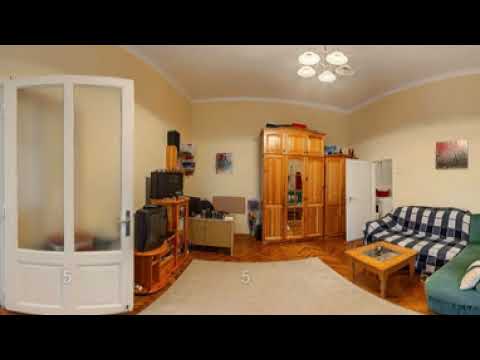The image depicts an indoor scene, resembling a college dorm room or a living room. The setting is framed with a medium-thick black border at the top and bottom, emphasizing the room's contrast. The floor is primarily brown parquet with a large beige carpet centrally placed. To the left, there's a white door marked with the number five. Moving inward, various items and furniture pieces clutter the space, resembling storage units with desks, filing cabinets, and a TV. A blurred-out picture is visible on the wall. Centered in the image, there's a tall freestanding wooden chest of drawers, flanked by another wooden cabinetry unit to its right. Further right, a white door potentially leading to a kitchen or laundry room is seen. A blue and white plaid couch sits adjacent, accompanied by a small coffee table. Above, five ceiling lights are present, but one appears blurred. The walls are beige, accented by a white ceiling, encapsulating the diverse arrangement of colors including black, white, brown, green, red, purple, orange, and yellow.